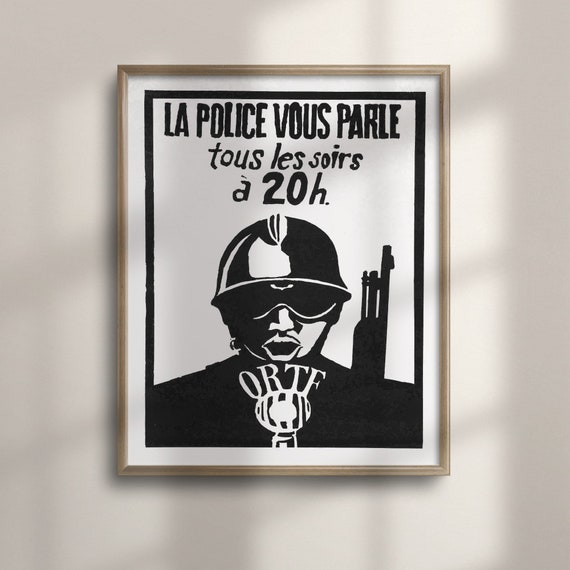The image captures a framed black and white French propaganda poster hanging on a white wall with a wooden frame. The poster itself features a secondary black frame within the main frame. At the top of the poster, French text reads, "La police veut parler de les soeurs à 20 heures," which translates to something akin to "the police will parley to this story at 20:00 hours." 

The central figure in the poster is a soldier or authoritarian figure, wearing a helmet and black glasses that obscure a portion of his face. His mouth is open, and he dons a black uniform. Emblazoned across his chest are the letters "ORTF," situated above a circular logo featuring bars that evoke an imagery akin to that of a prison. 

Also noticeable is the outline of a gun's barrel protruding from behind his shoulder to the right of his head. The wall behind the framed poster shows dynamic lighting, casting shadows, especially towards the right side, and there's a faint grid pattern over the surface, adding to the overall starkness and intensity of the scene.